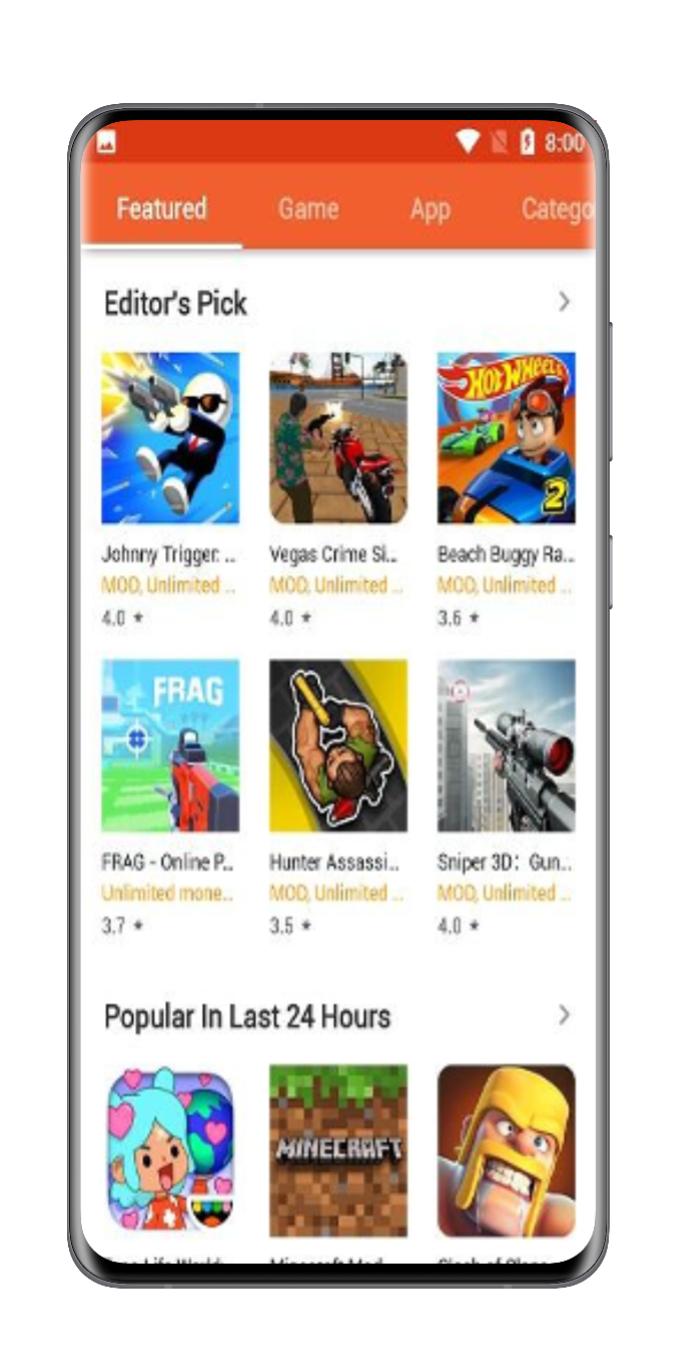A detailed depiction of a cell phone screen displays a black or dark gray border and a vibrant orange-red background. At the top, a small white square with orange zigzags is accompanied by an indication of the time, "8:00," on the right side. Adjacent to the time is a white battery icon with a lightning bolt, indicating low battery status, a partially faded battery with a line through it, and a clear white sound bar.

Centered at the top, text in white reads "Featured," "Game," "App," and "Category," with "Featured" being underlined. Below this header, there is an Editors' Picks section. Three rows of app names are displayed in columns. The first row includes "Johnny Trigger," "Vegas Crime," and "Beach Buggy RA." The second row features "Frag-OnlineP…," "Hunter Assassin," and "Sniper 3D Gun…," each adorned with small, cartoonish icons representing the respective apps.

Further down, black text identifies a section titled "Popular in Last 24 Hours." This section shows three images, though the left and right images are partially obscured except for recognizable elements. The middle image is identified as "Minecraft," while the far right image is of a cartoonish figure wearing a helmet, with a yellow mustache and large, white teeth. Another partially visible image is on the left.

Overall, the phone screen presents a vivid and organized display of popular games and editor’s picks for the user to explore.